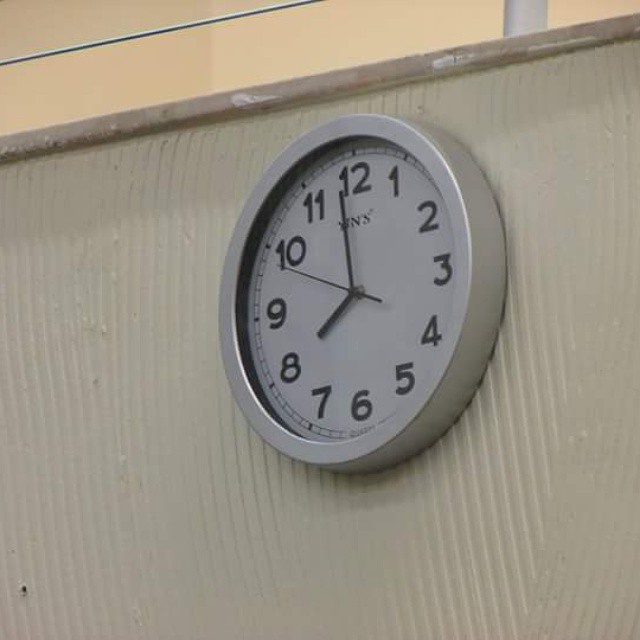The image depicts a silver clock with a stainless steel finish mounted on a tan-colored wall featuring a textured, ridged surface. The clock itself has a white face with three black hands: a thin, needle-like hand for the seconds, a long, slender hand for the minutes, and a shorter, broader hand for the hours. At the top of the wall, there is a thin wooden border. In the upper part of the image, a peach-colored wall is visible, adorned with a gray pipe in the right corner and a blue line running horizontally across the top.